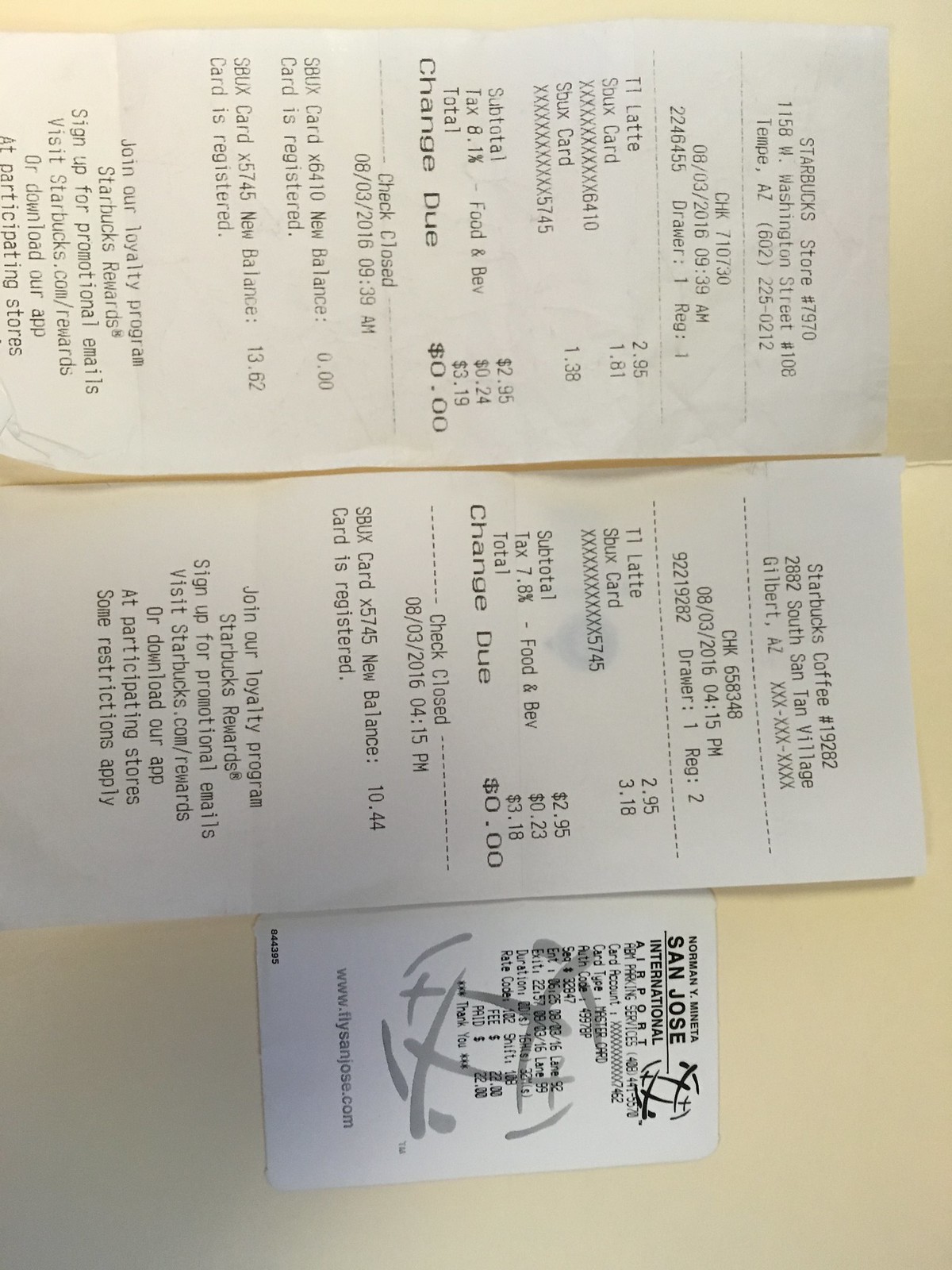This color photograph has been rotated 90 degrees clockwise, requiring one to tilt their head right to view it correctly. The composition consists of three receipts laid out on a yellow background. A visible crease runs between the first and second receipts, adding texture to the backdrop.

The first receipt, positioned at the top, is from Starbucks. It lists a total amount of $3.19 and indicates no change due. At the bottom, it states "check closed" followed by additional text that is not fully legible.

The second receipt, also from a Starbucks store but from a different location, resides directly beneath the first. The addresses on the receipts differ; the first address is 1158 W Washington St, #108, and the second is 22 South San Terry Village. This receipt also totals $3.18, with similar end text stating "check closed," but features only one line of text underneath, possibly indicating a discrepancy or error.

A third, smaller receipt is situated to the right of the Starbucks receipts. It is from San Jose International, bearing a prominent watermark—a circular object intersected by four lines, two vertical and two horizontal—obscuring some of the receipt's details including its total amount. A partially visible website address is printed at the bottom, though the text is too small to decipher. A smaller version of the watermark is also present at the top right corner of this receipt, contributing to the layered and intricate visual presentation.